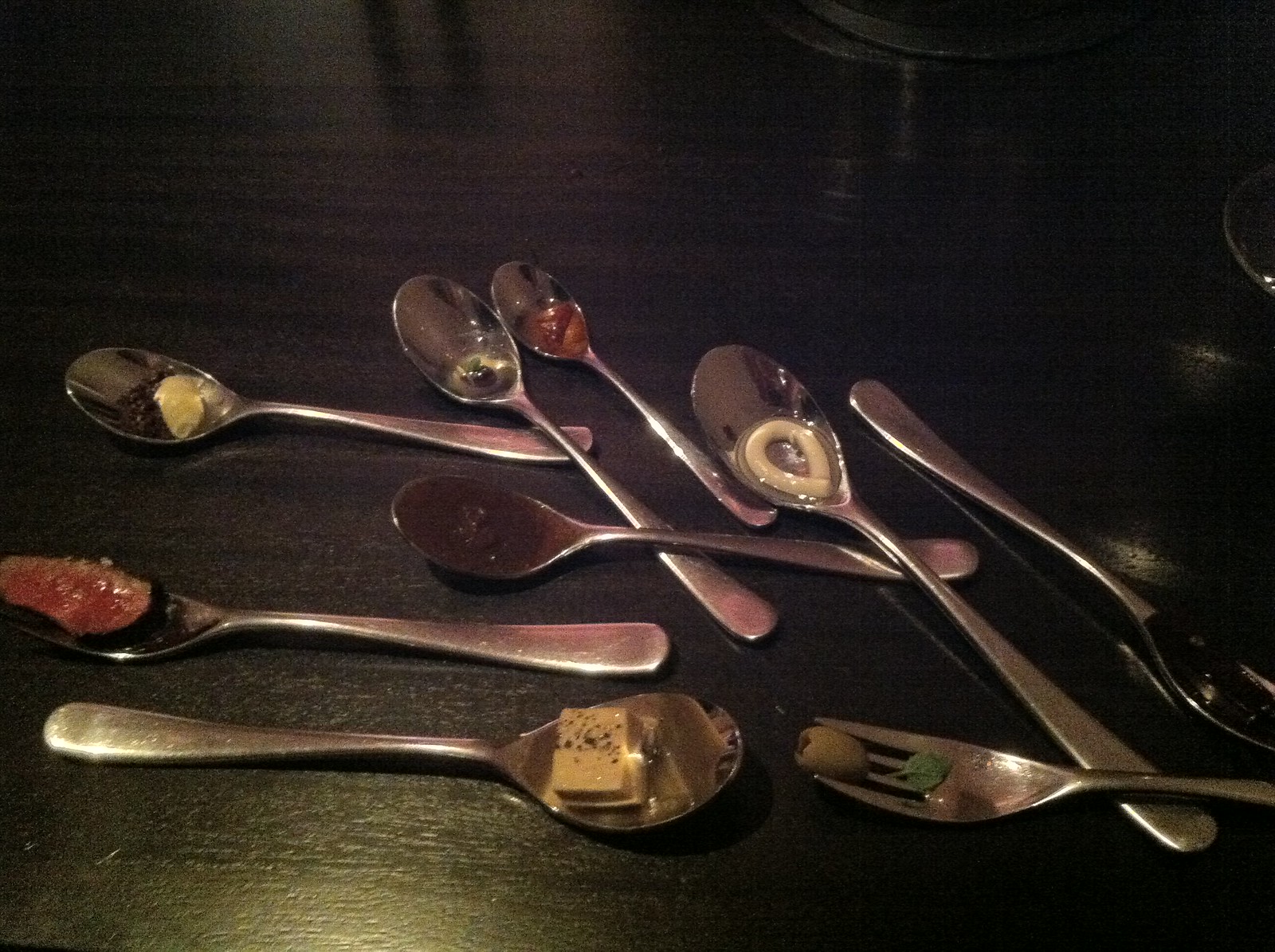The image depicts a set of eight silver or stainless steel spoons and one fork, all arranged on a dark, glossy wooden surface that resembles mahogany. Each utensil contains a different type of food, creating a diverse and intriguing array. The items in the spoons include a piece of meat, various sauces, what appears to be cheese, a noodle, and some indeterminate food slop. The fork is distinctively holding a green olive at its tip. The reflective surface of the table shows outlines or shadows, possibly of people, adding a subtle, ambient backdrop to the scene. Positioned on the right side of the frame is a glass bowl. The image, likely taken from a slight angle by the diner, captures the essence of a fine dining experience with international flavors.